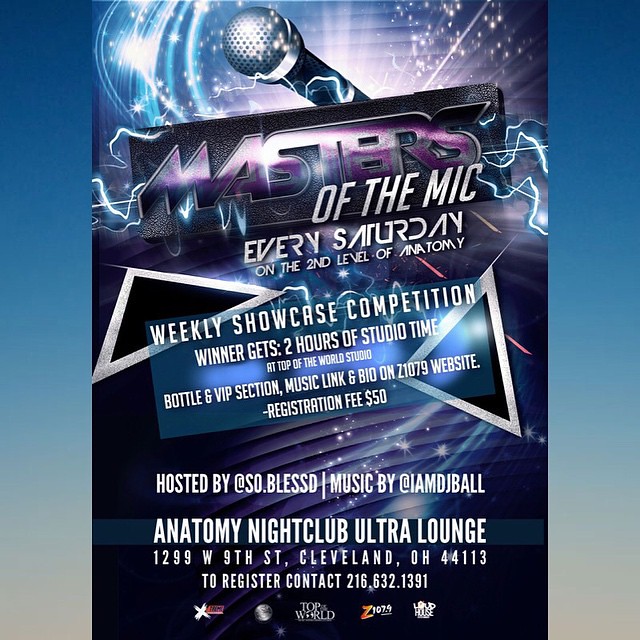The image is a dynamic advertisement for "Masters of the Mic," held every Saturday on the second level of Anatomy Nightclub Ultra Lounge at 1299 West 9th Street, Cleveland, Ohio 44113. The center of the image features a striking microphone emitting lightning bolts and blue streaks, adding to its energetic feel. The word "Masters" is prominently displayed in purple above a black bar, with "of the Mic" written in silver below it. The vibrant background, transitioning from blue to tan with sparkles, enhances the poster's lively atmosphere, complemented by side borders that fade from dark blue to gray. The advertisement details the weekly showcase competition, where winners earn two hours of studio time at Top of the World Studio, along with a bottle and VIP section. Information about the event includes a $50 registration fee, music by DJ Ball, and hosting by So Blessed. Additional elements feature logos for Z107.9, Loud House, and Top of the World, with further details, music links, and bios available on the Z107.9 website. To register, contact 216-632-1391. The overall aesthetic, dominated by blues, purples, and silvers, makes the advertisement visually compelling and informative.